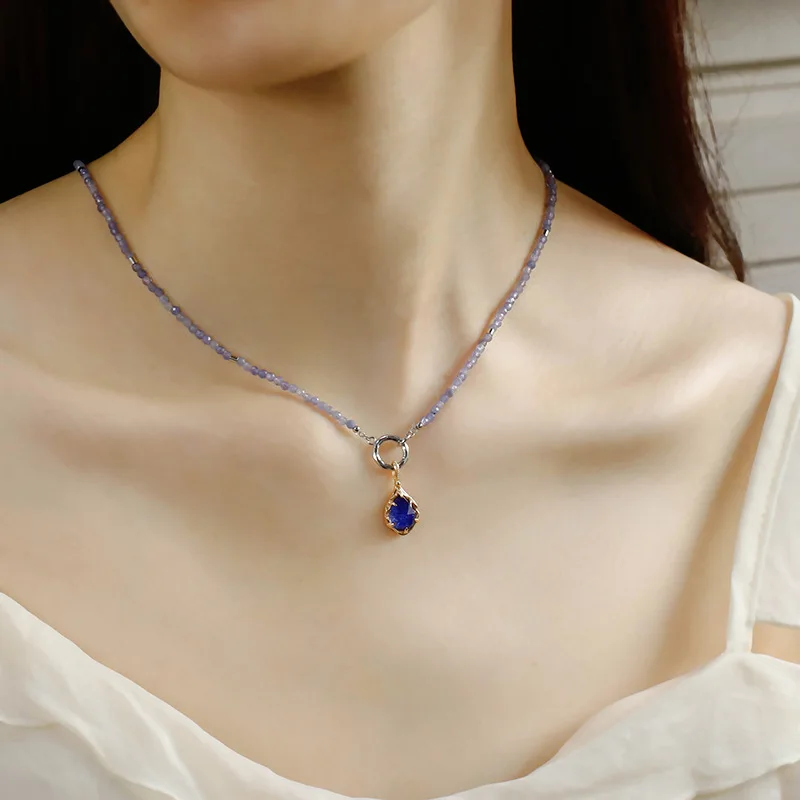This image captures a close-up view of a young Caucasian woman's neck and upper chest, showcasing her collarbone and the outline of her chin. She is wearing a low-cut white blouse, against which her very pale skin contrasts distinctively. Her dark brown hair falls behind her back, and the background appears to be a white wall with horizontal lines, possibly made of wood.

The focal point of the image is her intricate necklace. The necklace features a chain composed of small, varying shades of purple beads, giving it a delicate, handmade appearance. At the center of the necklace is a silver hoop, from which a stunning blue sapphire pendant delicately hangs. This deep blue gemstone is encased in a gold clasp, creating a beautiful blend of metals that enhances the necklace’s elegance. The detailed capture of her collarbone and the shadowing adds depth to the composition, emphasizing the intricate design and craftsmanship of the necklace.